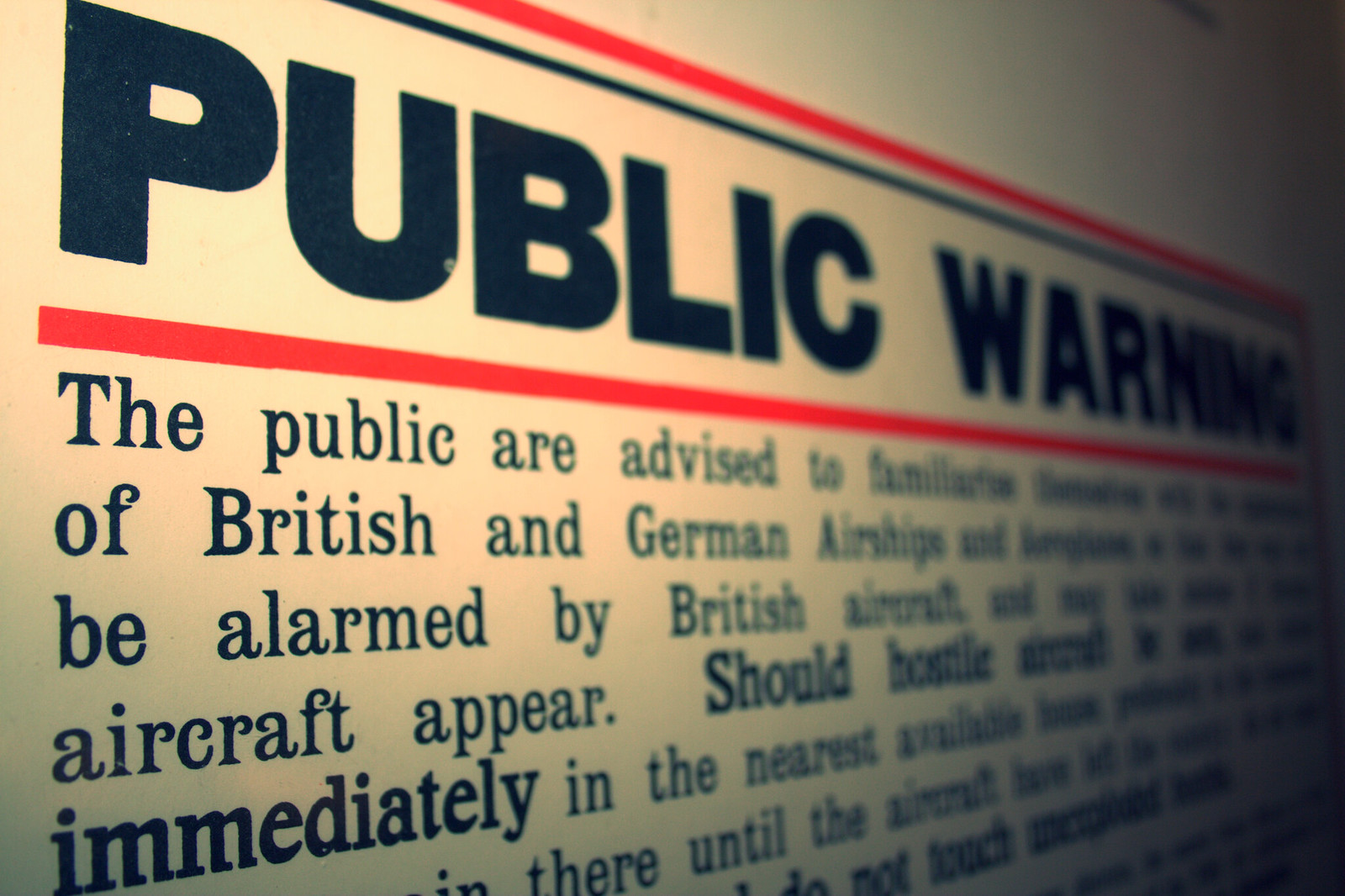This image captures a close-up of a public service announcement, possibly from a magazine, newspaper, or wall poster, which is slightly slanted. The announcement is characterized by a notable blur towards the right side, making some text difficult to decipher. Central to the image, the top half features a headline in large, bold, black text that reads "PUBLIC WARNING," flanked by two red horizontal rules above and below the headline. The more legible left side of the announcement begins with, "The public are advised to familiarize..." followed by partially readable lines that mention "British and German airships" and "be alarmed by British aircraft." Due to the blur, the further text is fragmented, with phrases like "aircraft may appear," and "should hostile," concluding with "immediately in the nearest available..." The overall tone and elements suggest a wartime warning message, with a palette that includes white, off-white, red, dark blue, and possibly gray hues.